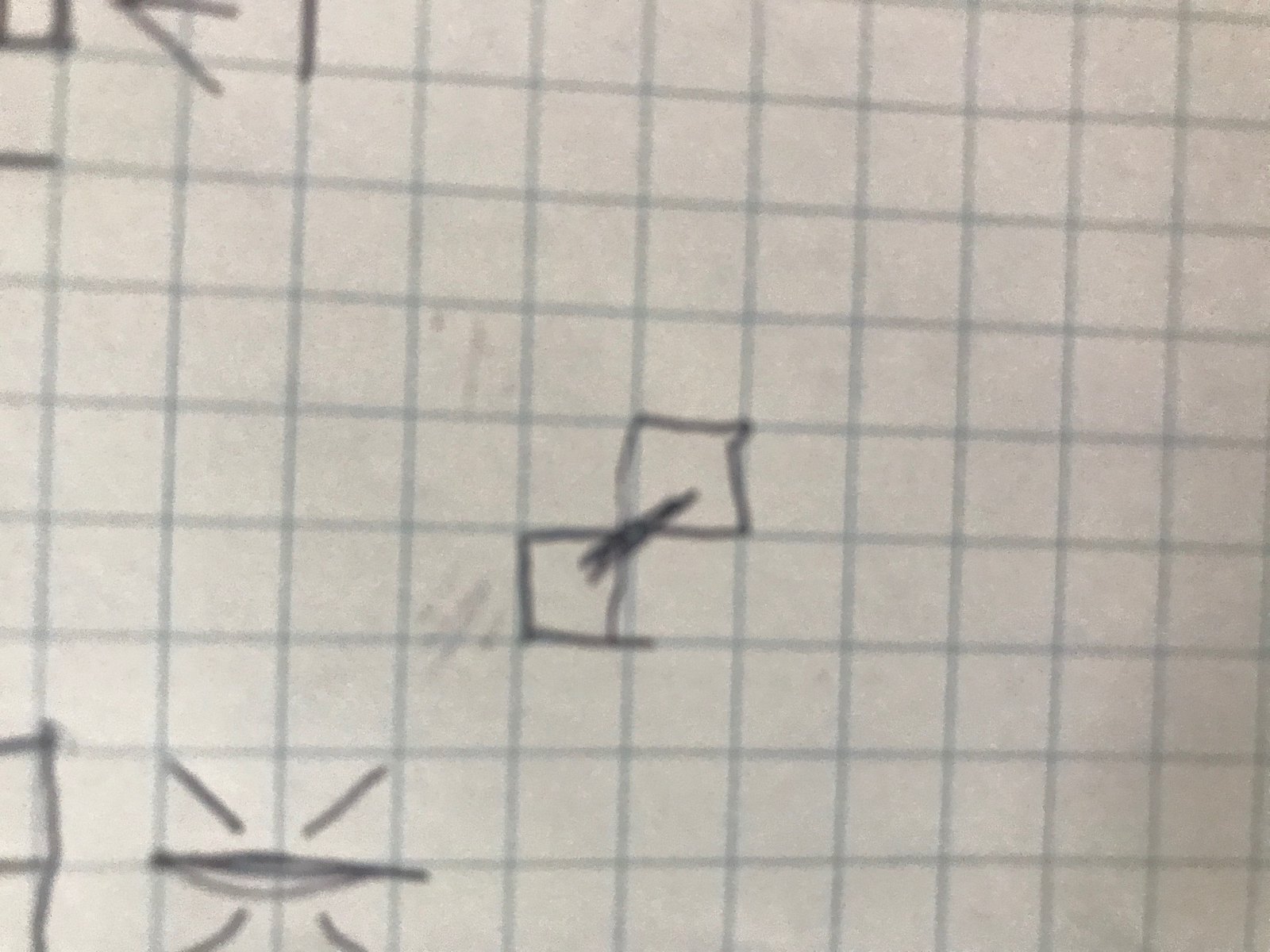Close-up of a piece of well-used, slightly grungy graph paper. The white paper features a blue grid and shows various pencil marks, including two adjacent squares filled in and connected by a line, suggesting a game of Battleship. In the bottom left corner, a horizontal line spans two squares, with diagonal lines in the four surrounding squares. Additional outlined squares and indistinct pencil marks are visible in the top left area, adding to the indication of a Battleship game in progress. The paper appears thin, with some bleed-through or ghost images, possibly from darker ink or illustrations beneath or on the reverse side. Light eraser marks and the overall worn appearance suggest multiple use, enhancing the authenticity of a spontaneous, hand-drawn game session.